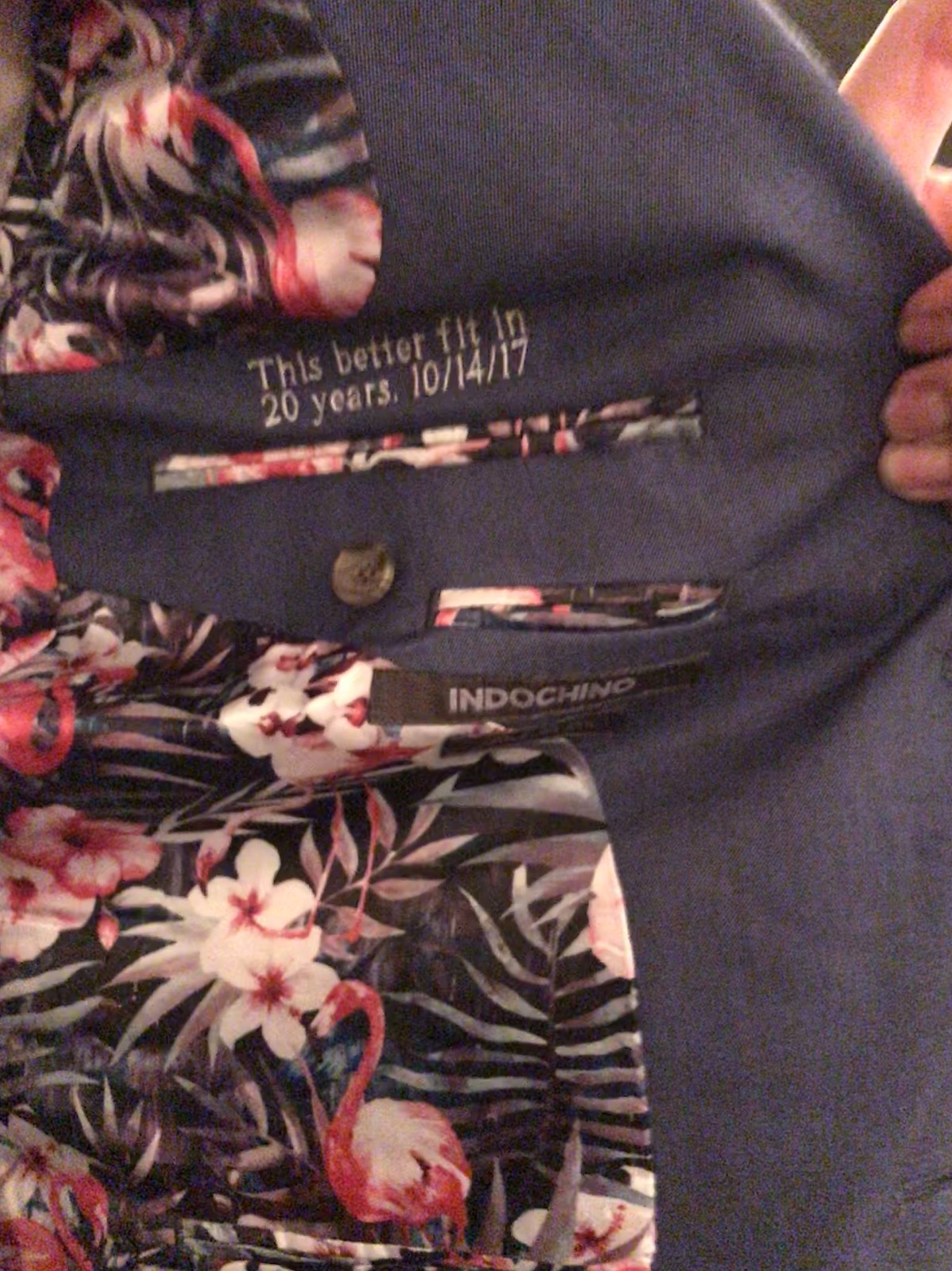A person's hand and part of their arm emerge from a dark background, holding a garment—a pair of gray pants with a visible button on the back pocket. The waistband features a label that reads "Indochino" with white lettering stating "This better fit in 20 years" dated 10/14/17. Additionally, draped over the arm is a vibrant shirt adorned with a pattern of black leaves, white flowers with pink centers, and pink flamingos, adding a pop of color against the dark backdrop.